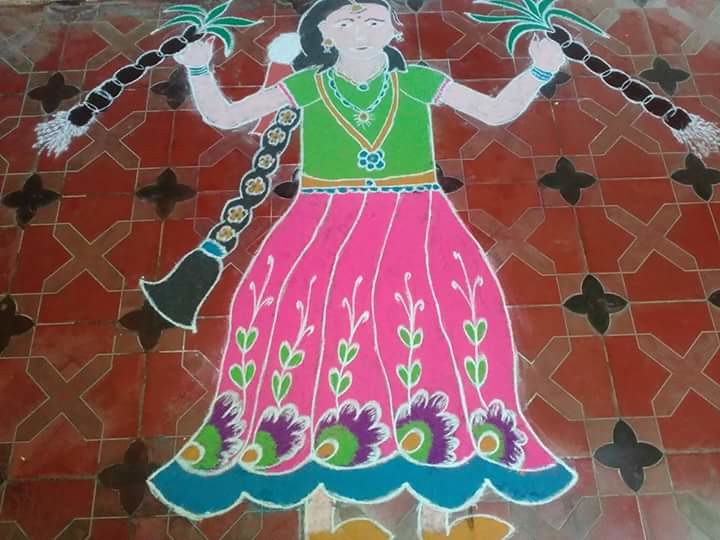The image portrays a vibrant floor painting of a woman, possibly of Indian or Mexican heritage, which is richly detailed and colorful. The woman is dressed in a green short-sleeved t-shirt and a pleated long pink skirt adorned with intricate designs resembling peacock feathers and floral patterns. Her hair is styled in a long, intricately braided ponytail decorated with small flowers. She is accessorized with multiple necklaces and bracelets. In her hands, she holds two miniature trees with green leaves, possibly palm trees, raised up in the air. She has yellow shoes on, with her feet pointing to the right. The painting lies on a red platform that features an array of light red X's and black clove-like designs, adding further detail to the artistic floor composition.